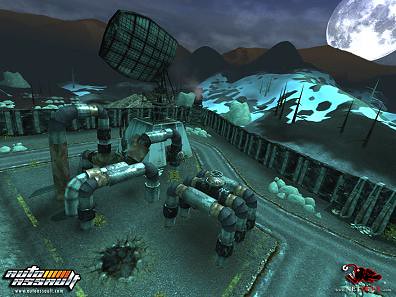In this in-game screenshot from "Auto Assassin," the player navigates through an industrial landscape. The bottom left corner displays the game's title in prominent white font. The scene reveals a paved gray ground with intricate pipework at its center. Half-circle pipes, accented with silver, gold, and black hues, tunnel into the ground, flanked by a square metal structure. The area is enclosed by a fence on both sides, leading to a backdrop of rugged brown mountains capped with patches of white snow. The sky above is partly cloudy, featuring a large, bright full moon in the upper right corner. A satellite-like structure stands at the center of the image, adding to the tech-industrial ambiance. Sparse, leafless trees dot the snowy hillside, enhancing the desolate, yet intriguing, atmosphere of the game environment.